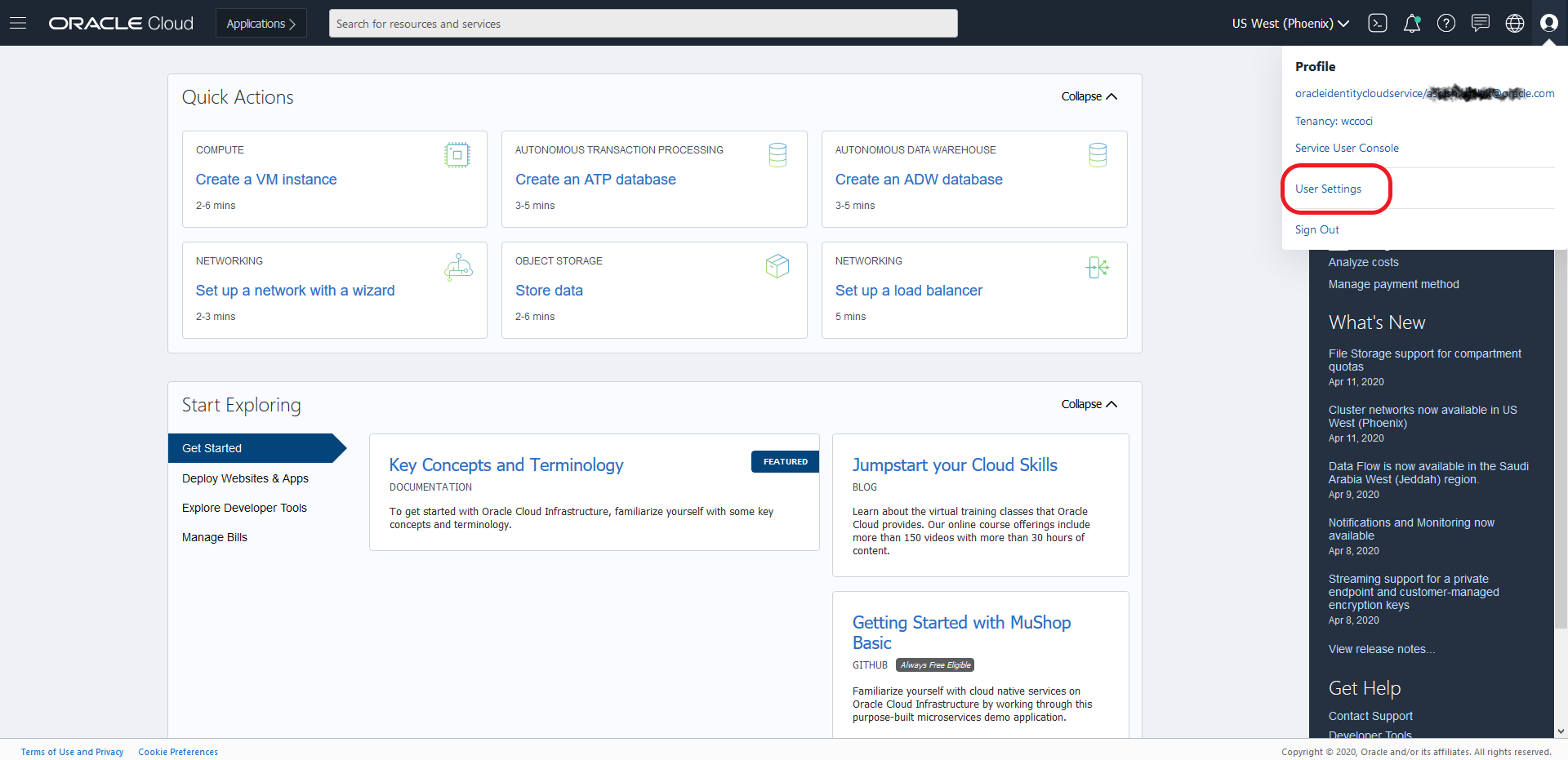The image displays the Oracle Cloud website interface, characterized by its clean, professional layout and striking navy blue color theme. A navy blue banner stretches across the top of the page. On the upper left-hand corner of this banner, there are three parallel lines indicating a menu button. Next to this, the "Oracle Cloud" logo is prominently displayed in white font. Adjacent to this, there's an option that appears to read "Applications." Following this, towards the center-right, there's a search field. To the far right of the search field, a set of icons is present, which potentially includes a notification icon and an account icon, though their details are too indistinct to discern clearly.

Below the banner, the first section is titled "Quick Actions." This section contains six distinct boxes, each representing different quick action options available for selection. On the far right side of this section, there's a collapse button that allows users to hide the "Quick Actions" area.

Beneath the "Quick Actions" section, there's another area named "Start Exploring." This section is divided into two parts: the left side lists several options for exploration, though the text is too small to read. The topmost option in this list is highlighted with a blue square, indicating it is the selected choice. Right next to this, on the right side, there's a box labeled "Key Concepts of Terminologies."

Further down the page, on the right side, there's a "Profile" section with four to five options. The option labeled "View Settings" is marked conspicuously with a red circle.

At the bottom of the image, a "What's New" section stands out with its dark navy blue background, and white and blue font, drawing attention to recent updates or features.